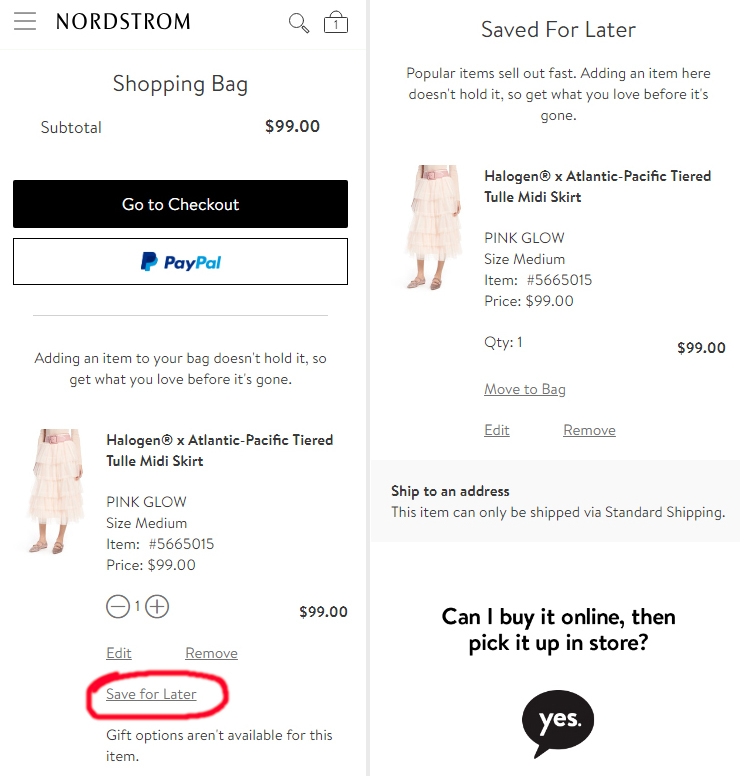Screenshot of the Nordstrom Shopping Cart Checkout Page

The interface features a clean, white background. At the top left corner, there are three horizontal dark gray lines, representing a menu. To the right of these lines, the word "NORDSTROM" is displayed in bold, black, all-caps text. Adjacent to the text, there's some negative space leading to a black magnifying glass icon followed by a shopping bag icon containing the number 1, indicating one item in the cart.

Below this header, a thin gray line spans across the page, under which the words "Shopping Bag" are centered in black text. Below this title, on the left side, light gray text displays "Subtotal," while bold black text on the right side shows "$99."

Directly underneath, a black button with white text reads "Go to Checkout." Below this, a white button with a black outline contains the word "PayPal" in blue text, with "Pay" in dark blue and "Pal" in light blue. To the left of the PayPal text, two overlaid Ps appear, with the top P in darker blue and the bottom P in lighter blue.

Following this, there's a slightly thicker light gray line, below which a light gray notice reads, "Adding an item to your bag doesn't hold it, so get what you love before it's gone."

Towards the bottom left of the page is an image of a woman wearing a pink, tiered tulle midi skirt. To the right of the image, gray text describes the item as "Halogen ex-Atlantic-Pacific Tiered Tulle Midi Skirt." Below this description, additional gray text lists the color as "Pink Glow," the size as "Medium," the item number as "5665015," and the price as "$99."

Beneath the product details, a quantity selector displays the number "1" flanked by a minus sign on the left and a plus sign on the right, with the total price of "$99" bolded to the right. Additional product information is repeated and elaborated on the right side of the page.

The interface provides a thorough and visually organized summary of the shopping cart contents, complete with intuitive navigation and payment options.